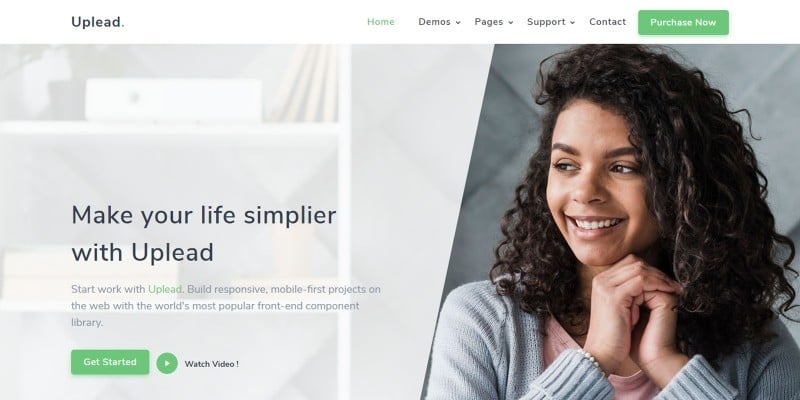In the image, the top navigation bar features options such as "Uplead," "Home," "Demos," "Pages," "Support," "Contact," and "Screens," which appear to indicate the sections of the website. The slogan "Make your life simpler with Uplead" is prominently displayed, encouraging users to start using Uplead. A description follows, touting Uplead's ability to help users build responsive, mobile-first projects on the web using the world's most popular front-end compatible library.

Below the slogan, there is a green rectangle button labeled "Get Started," inviting users to begin their experience with Uplead. Adjacent to this button, there is a green circle featuring a play button icon, prompting users to watch a video.

On the right side of the image, a woman with curly dark hair is depicted. She stands in a light-colored background, wearing a white sweater layered over a pink shirt, with a grey garment visible underneath. She appears to have one hand resting on the other, adding a personable and approachable element to the presentation of the website. The overall design suggests a welcoming, user-friendly experience for those interested in utilizing Uplead's front-end library services.